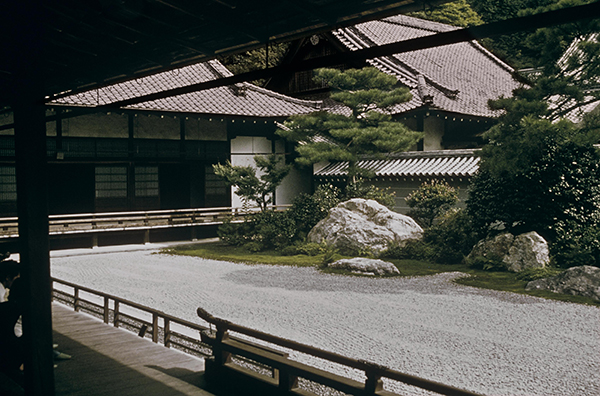The image is a serene, wide view shot of a traditional Japanese architecture compound, seen from within a shaded, roofed outdoor area. The driveway, lined with white gravel, leads into the heart of the compound. To the left, part of the structure is visible, showcasing a traditional Japanese style roof, white paneled walls with wood accents, and a silver rail in front. On the right side, another section of the structure appears with a separate roof and a wall in front. The right side of the driveway is meticulously landscaped with large boulders, beautiful plants, and little bonsai trees, adding to the tranquil ambiance. The mid-ground features a graveled courtyard adorned with large rocks and bonsai trees, with the building wrapping around from where the viewer stands. The overall architecture is dark wood with white highlights, steep roofs, and tiled accents, giving a peaceful and beautiful effect. The scene's lighting suggests it is either dusk or a possibly cloudy daytime, with a forest visible in the background against the highest roof, evoking the atmosphere of a traditional tea house or palace setting.